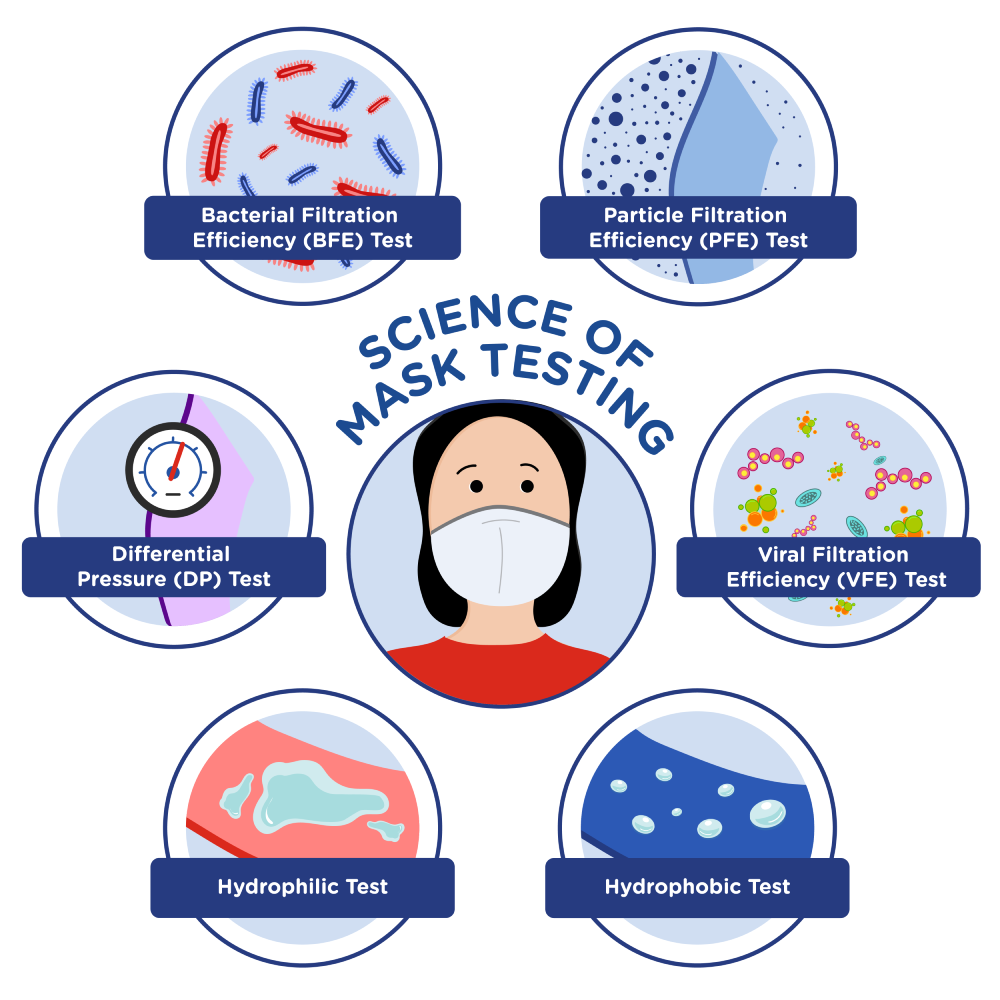The image features a simple cartoon drawing of a woman with black hair, wearing a white face mask and a red shirt, depicted in a central circle with a dark blue outline. Above the woman, in capitalized blue text, it reads "SCIENCE OF MASK TESTING." Surrounding the central circle are six smaller circles positioned like the hours on a clock: two on top, one on each side, and two on the bottom.

Each of these outer circles contains an illustration and a blue banner with white text detailing a specific mask test. Starting from the top right and moving clockwise:
1. **Particle Filtration Efficiency (PFE) Test**: Shows large blue particles on the left and smaller particles on the right after passing through a filter.
2. **Viral Filtration Efficiency (VFE) Test**: Illustrates pink and blue microbes.
3. **Hydrophobic Test**: Features water droplets on what appears to be a sponge, demonstrating water resistance.
4. **Hydrophilic Test**: Depicts water spreading out on a pink fabric, indicating absorbency.
5. **Differential Pressure (DP) Test**: Presents a gauge with a red needle pointing at one o'clock.
6. **Bacterial Filtration Efficiency (BFE) Test**: Shows red and blue microbes.

The background of the image is plain white, enhancing the vividness of the illustrations and text. This detailed layout emphasizes the different types of filtration and resistance tests masks undergo.